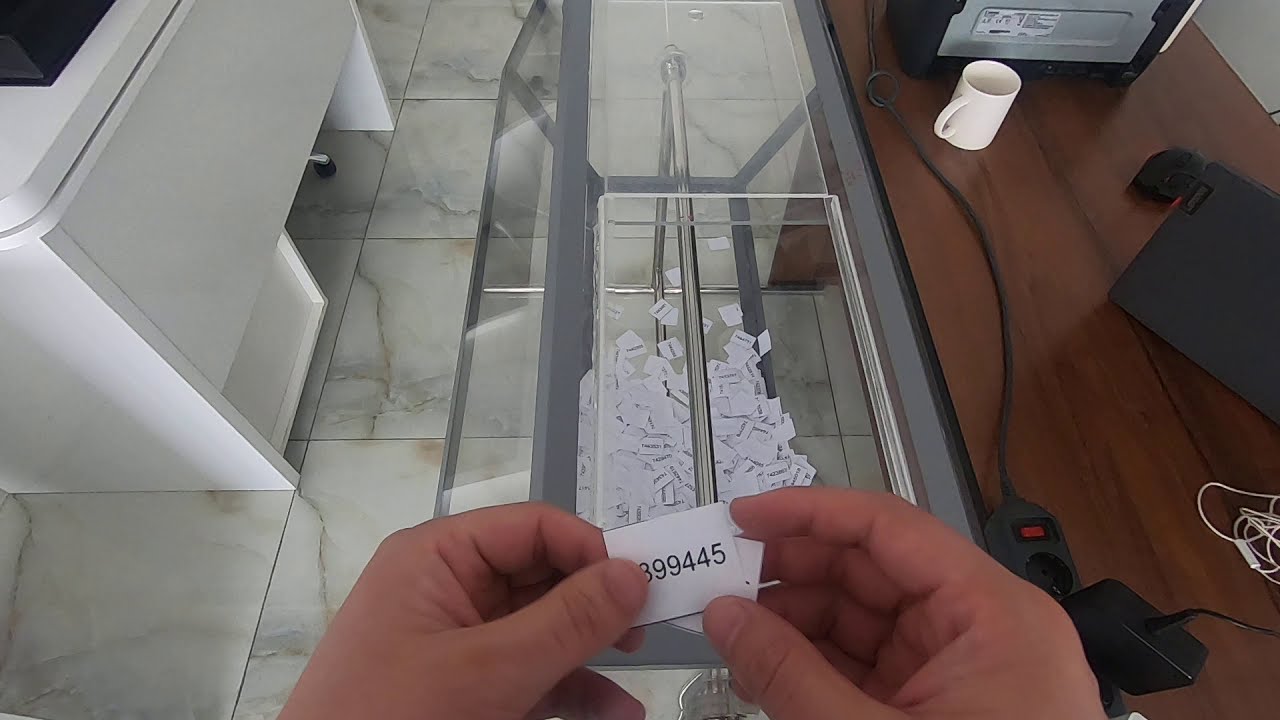In the horizontally aligned rectangular image, the focal point is a pair of hands positioned at the bottom center, holding a small rectangular piece of white paper with the black numbers "399445" on it. Below the hands, there is a transparent plastic container teeming with similar numbered pieces of paper, reminiscent of a raffle or lottery system. To the right, a brown desktop hosts a white coffee mug, a black surge protector with a red toggle switch, and various cords including a coiled white one. On the left, the floor is covered with white marbled tiles. Near the upper left corner, a white desk or countertop can be seen with a black object partially visible atop it.